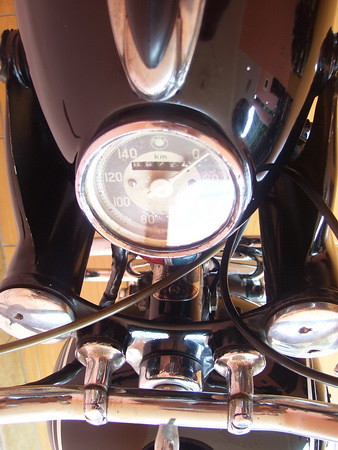This vertical rectangular photograph showcases a detailed close-up of a circular dial resembling a speedometer. The speedometer has a silver bezel encircling the dial, which darkens at the top. The numbers on the dial are visible but partially obscured by bright light reflecting off the surface. At the position where one o'clock would be on a clock face, the dial displays '0.' The bright glare obscures the numbers until the 7 o'clock position, where '80' is visible. Continuing around the dial, '100' appears at 8 o'clock, '120' at 9 o'clock, and '140' at approximately 10 or 11 o'clock. At the 12 o'clock position, there's a distinctive white circle, beneath which lies a black counter that appears to display numbers, although they are unreadable in the photograph.

The center of the dial features a white circular section with a white needle pointing to just past the '0', near the 1 or 2 o'clock mark. The dial is set within a dark metal structure, possibly part of a motorcycle or a moped, suggesting that the photograph may be oriented upside down. The upper body of the vehicle, therefore, appears at the top of the image.

Emerging from around the dial are several black wires. One wire extends to the left-hand side about two-thirds of the way down, another runs from the center to the bottom right corner, and a third wire leads to the middle of the right side.

At the bottom of the photograph, a horizontal bar spans from the lower left to the lower right side, intersected by two smaller vertical bars positioned equidistantly from the horizontal bar. These vertical bars flank a large silver rectangular piece located in the center. Above these vertical bars are two circular pieces with silver tops, which are slightly obscured by glare. These circular components are connected to a black structure extending from just below the middle of the right and left sides, reaching towards the upper left and upper right corners.